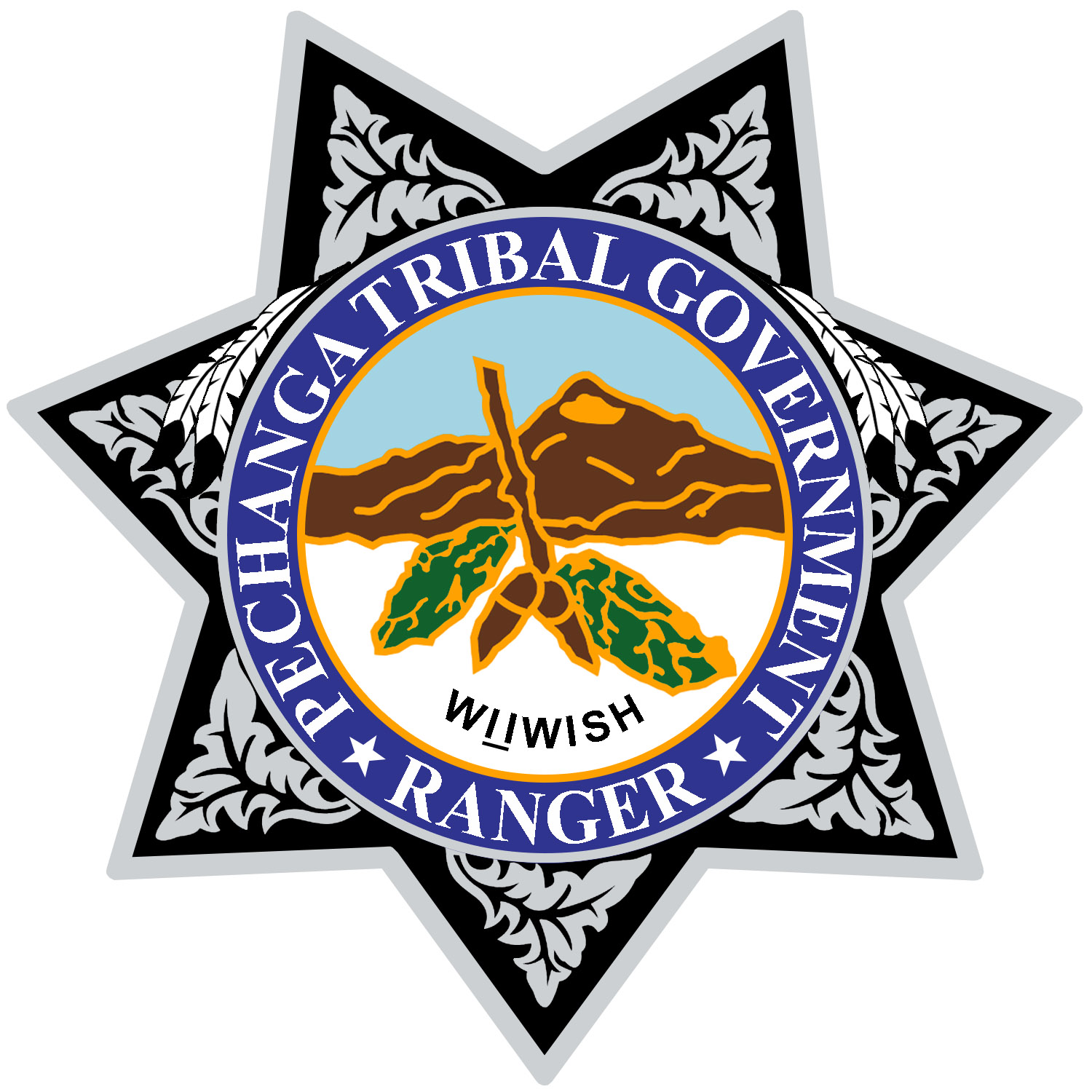This is a detailed illustration of a seven-pointed star badge against a white background. The badge has a decorative black and gray design, featuring a gray border and a patterned gray leaf design within each of the star’s points, set against a black background. Surrounding a large central circle are two feathers positioned on either side. The central circle has a thick blue border with white lettering that reads "Pechanga Tribal Government," accompanied by a small white star before "Pechanga" and after "Government," and the word "Ranger" at the bottom. Inside the circle, a light blue sky forms the backdrop for a detailed scene, including brown mountains shaded with darker brown, and a brown branch with green leaves framed by yellow borders. Below the mountains, the word "WIIWISH" is inscribed in black, with the I's underlined.